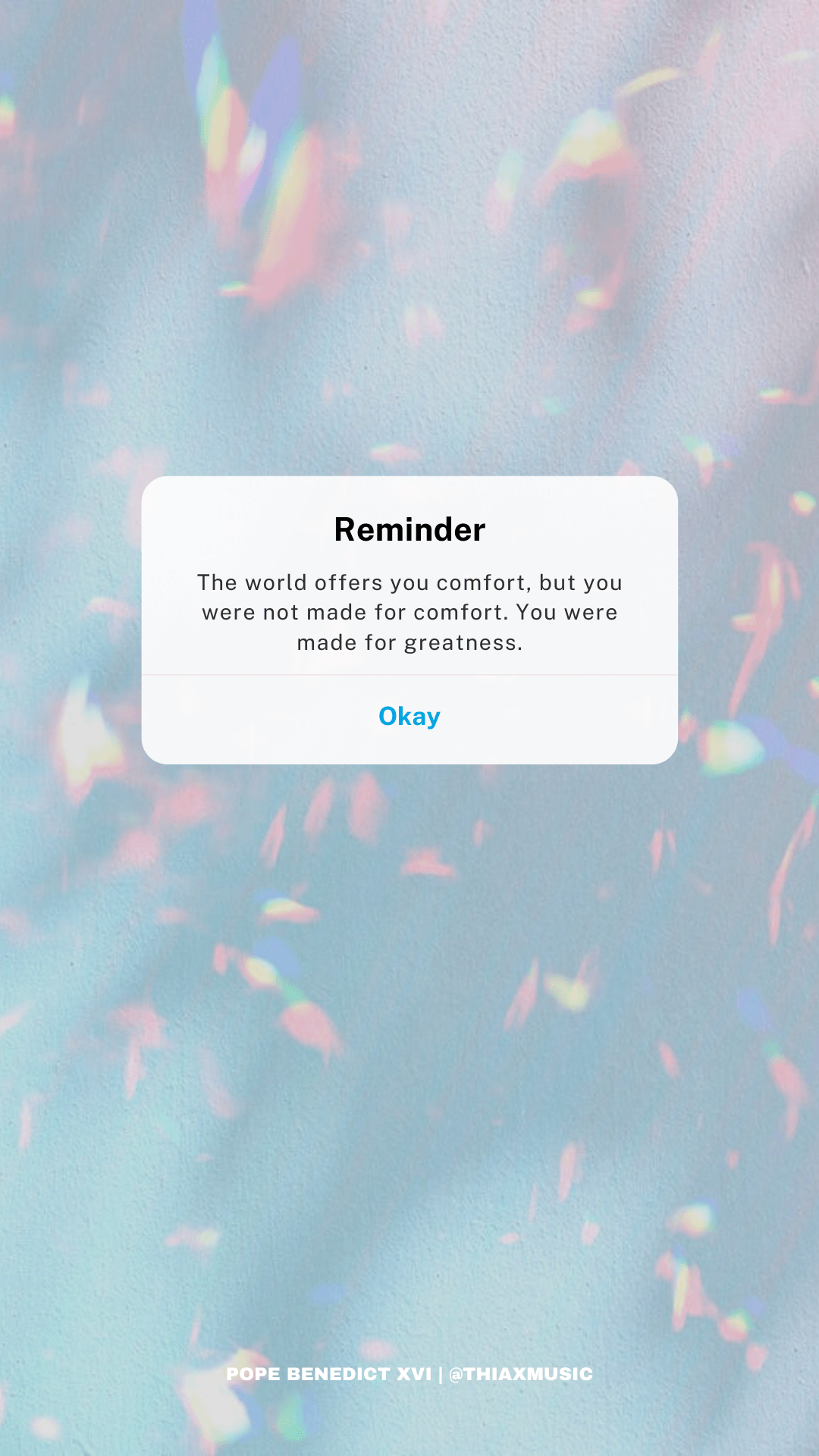This is a screenshot of a notification pop-up on an iPhone, situated slightly above the center of the screen. The notification is a white rectangle with rounded corners. At the top center of the pop-up, bold black text reads "Reminder." Directly below this, in thin, small gray text, it displays the quote: "The world offers you comfort, but you were not made for comfort, you were made for greatness." 

Near the bottom quarter of the pop-up, there is a gray dividing line with the word "Okay" in blue text centered beneath it. The pop-up is set against a backdrop featuring an abstract, light pattern with a ruffled texture. This background has a very light bluish-gray tone, accentuated with subtle rainbow-like colors scattered across its surface.

At the bottom of the screen, written in white, all-caps, sans-serif text, it says "Pope Benedict XVI." This text is separated by a white line from the phrase "At Thiax Music" positioned to the right. The remaining screen space is occupied by the aforementioned abstract background with no additional pop-ups or elements visible.